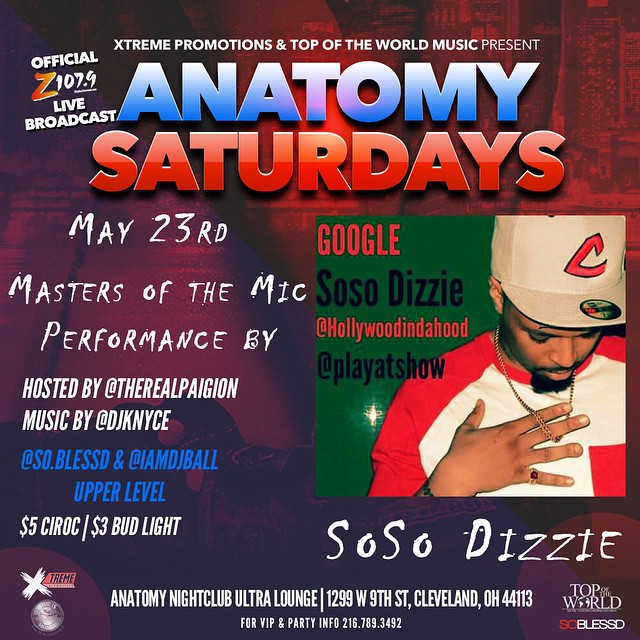The image is a vibrant, square poster advertising a rap concert event titled "Anatomy's Saturdays" at Anatomy Nightclub Ultra Lounge in Cleveland, Ohio. The background features a blend of green, reddish, and purple hues. Highlighted on the right side is a prominent picture of the entertainer, So So Dizzy, donning a red and white shirt and a Cleveland Guardians hat. The event, hosted by DK and YCE, is presented by Extreme Promotions and Top-of-the-World Music, and scheduled for May 23rd. Attendees can enjoy $5 Chirac and $3 Bud Lights. All essential details, including the nightclub's address (1299 West 9th Street, Cleveland, Ohio, 44113) and contact number (216-783-3492) for VIP and party information, are provided at the bottom in white text.